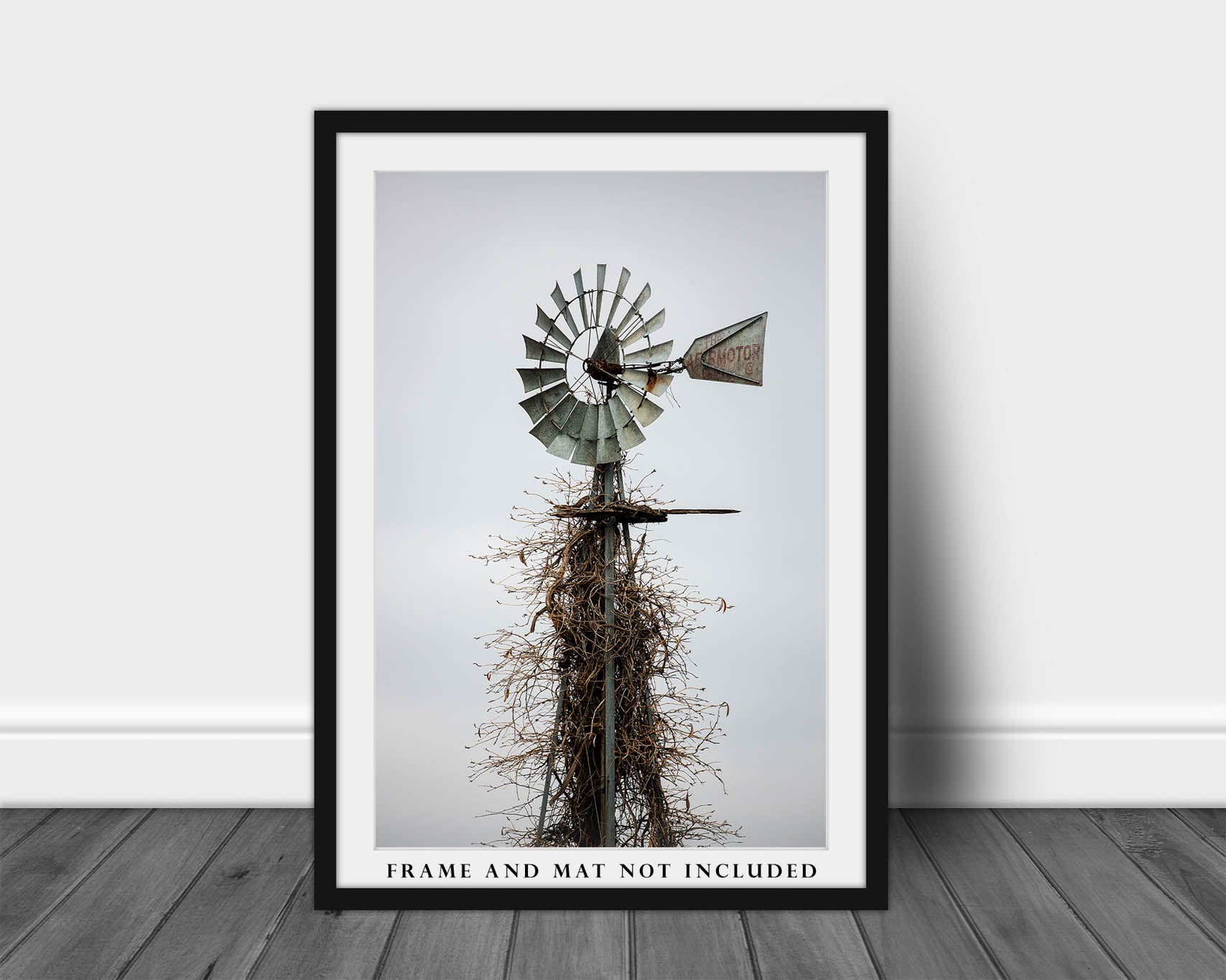This detailed photograph captures a framed black-and-white image of a rustic windmill, set against the backdrop of a white wall and gray hardwood flooring. The frame, a sleek black rectangle with a white matting, leans against the wall, centrally positioned in the image. Inside the mat, the windmill's blades face the camera while its tail points to the right, showcasing an emblem in sepia tones. Over time, old brown vines have climbed the windmill's metal masts, adding a touch of natural decay and history. A watermark at the bottom reads "frame and mat not included," indicating the image is a product example. The style of the photograph is realistic, emphasizing the textures and tones of the scene.